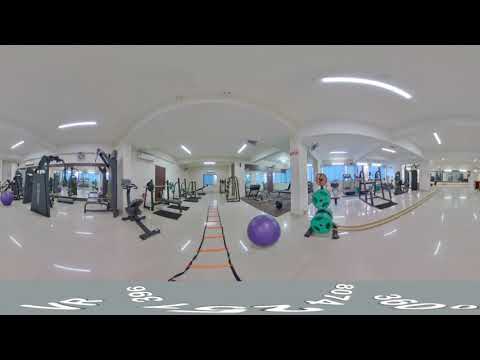This image presents a detailed panoramic view of a virtual reality gym setting, framed by a solid black border. The gym floor is a shiny white surface reflecting the ceiling lights above. The scene unfolds indoors during the day, featuring various pieces of exercise equipment. Centered in the foreground is a large purple exercise ball, surrounded by treadmills and walking machines aligned on either side of a central walkway leading to a blue door at the back. To the right, an expansive glass wall offers a glimpse of the blue sky outside. The left side of the room similarly showcases large windows. The gym includes intricate weight machines and additional exercise balls. Notable details such as the black, gray, white, light blue, purple, and green hues dominate the color palette. At the bottom of the screen, VR-related text and numbers (360, 8074) highlight this as an animated representation within a virtual reality environment.